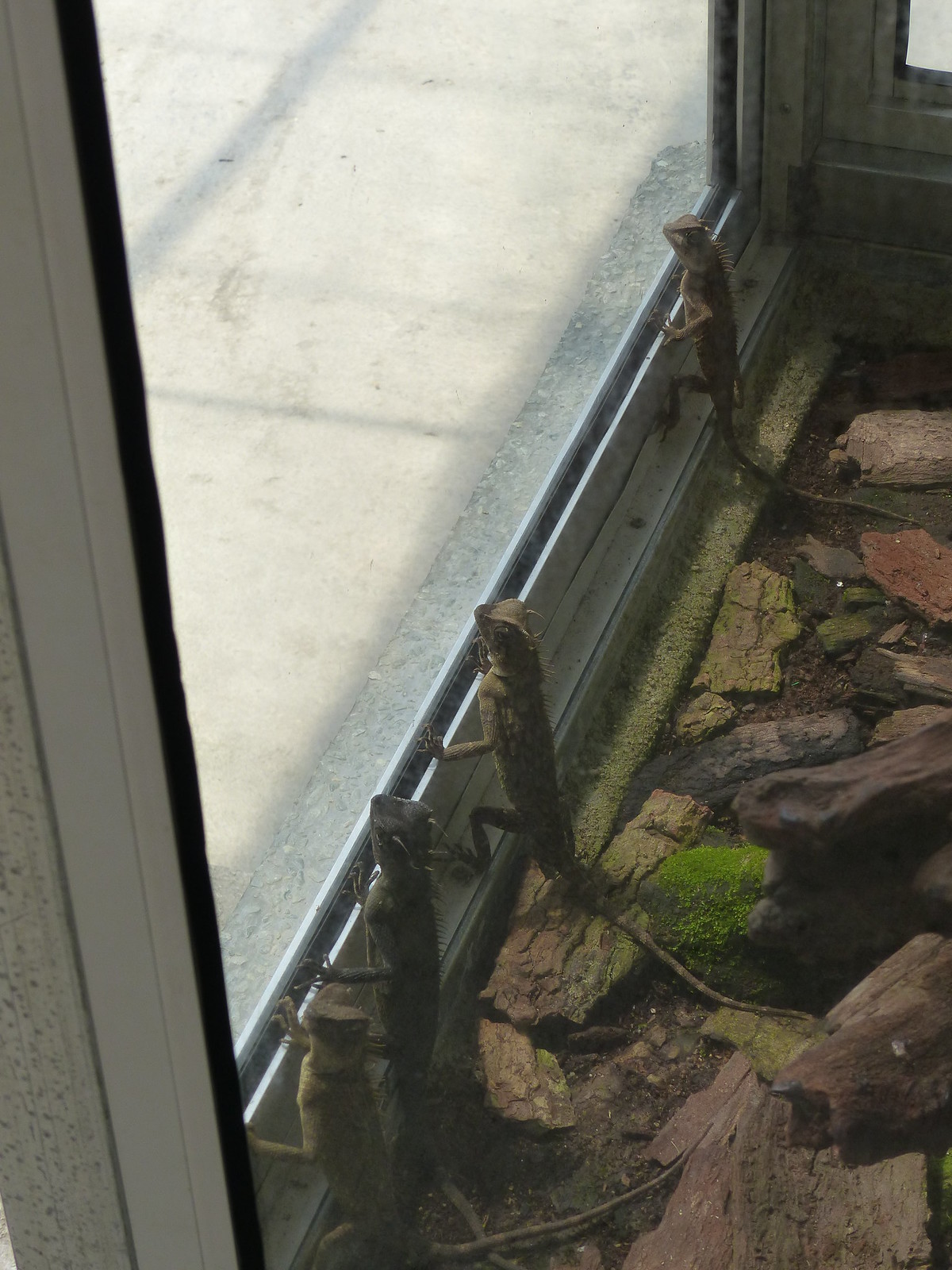The photograph captures a striking scene of four lizards, possibly baby iguanas, aligned diagonally from the bottom left to the top right, eagerly peering out through a glass patio door. The lizards, sporting a mix of greenish-brown hues with distinctive yellow spines running along their backs, stand on their hind legs with their front feet perched on the edge of the glass. Their tails extend straight out behind them while their back legs remain bent. One of the lizards has turned its head to look at the photographer, adding a touch of curiosity to the tableau.

They appear captivated by the view outside, where the daylight reveals a concrete sidewalk, although the scene beyond the glass remains somewhat ambiguous. The doorframe, with its white and slightly dirty borders, encases the glass pane, which is supported by a silver frame along the bottom and sides.

The lizards are positioned in their naturalistic enclosure, which features a rustic mix of moss, green patches, rocks, old logs, and sticks adorned with bits of lichen. The bark is predominantly brown with specks of green, creating a habitat that looks clean and well-maintained. The sunlight filtering through hints at a bright, inviting day outside, further highlighting the lizards' apparent longing to explore beyond their confined space.